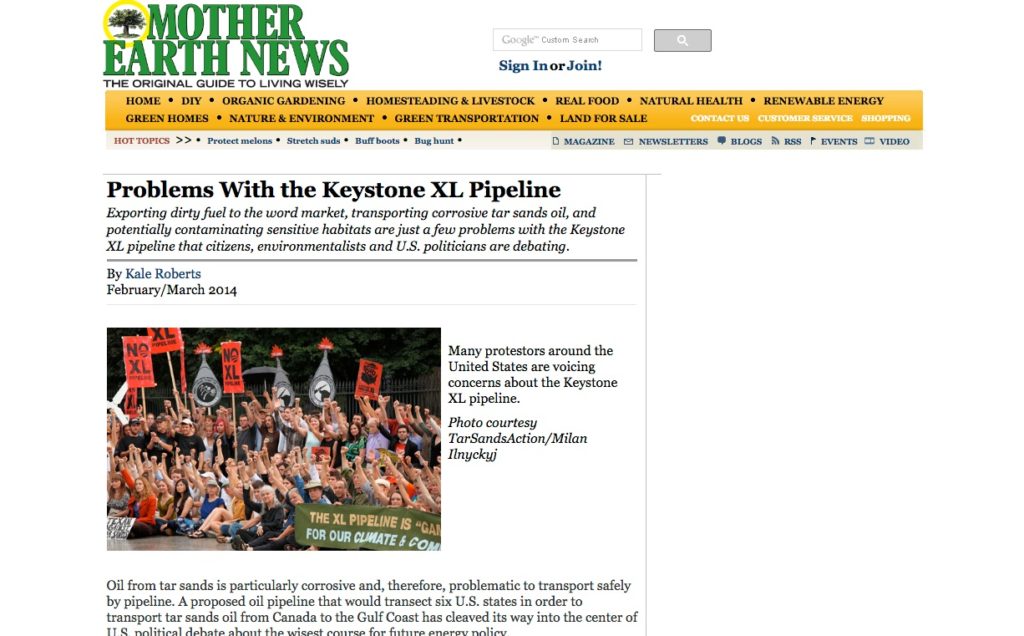This screenshot from the website "Mother Earth News" captures a detailed view of the site's home page. In the upper left-hand corner, the website's logo features the text "Mother Earth News" written in two lines, with a stylized tree enclosed in a yellow circle next to the word "Mother." Below the logo, the tagline reads "Original Guide to Living Wisely." To the right of the logo, there are options for users to "Sign In" or "Join."

The site has an orange background and includes two rows of menu options: 

- **First Row**: Home, DIY, Organic Gardening, Homesteading and Livestock, Real Food, Natural Health, Renewable Energy, Green Homes, Nature and Environment, Green Transportation, and Land for Sale. 
- **Second Row**: Contact Us, Customer Service, Shopping, Hot Topics, Protect Melons, Stretch Suds, Buff Boots, Bug Hunt.

Below the menu, additional options are provided: Magazine, Newsletters, Blogs, RSS, Events, and Video.

The focal point of the screenshot is an article titled "Problems with the Keystone XL Pipeline." The article discusses the contentious issues surrounding the pipeline, such as exporting dirty fuel to the world market, transporting corrosive tar sands, and the potential contamination of sensitive habitats. It highlights the debates among citizens, environmentalists, and U.S. politicians regarding these problems.

Accompanying the article is a photograph of a protest against the Keystone XL Pipeline. The image features a group of mostly women, some sitting and some standing, all holding signs that say "No XL" and raising their right fists in the air. The caption under the photograph states, "Many protests around the United States are voicing concerns about the Keystone XL Pipeline," mirroring the sentiment of the article.

The detailed content in the caption encapsulates the robust information and navigation structure of the "Mother Earth News" homepage, providing an extensive snapshot of current environmental issues and the community's engagement with them.